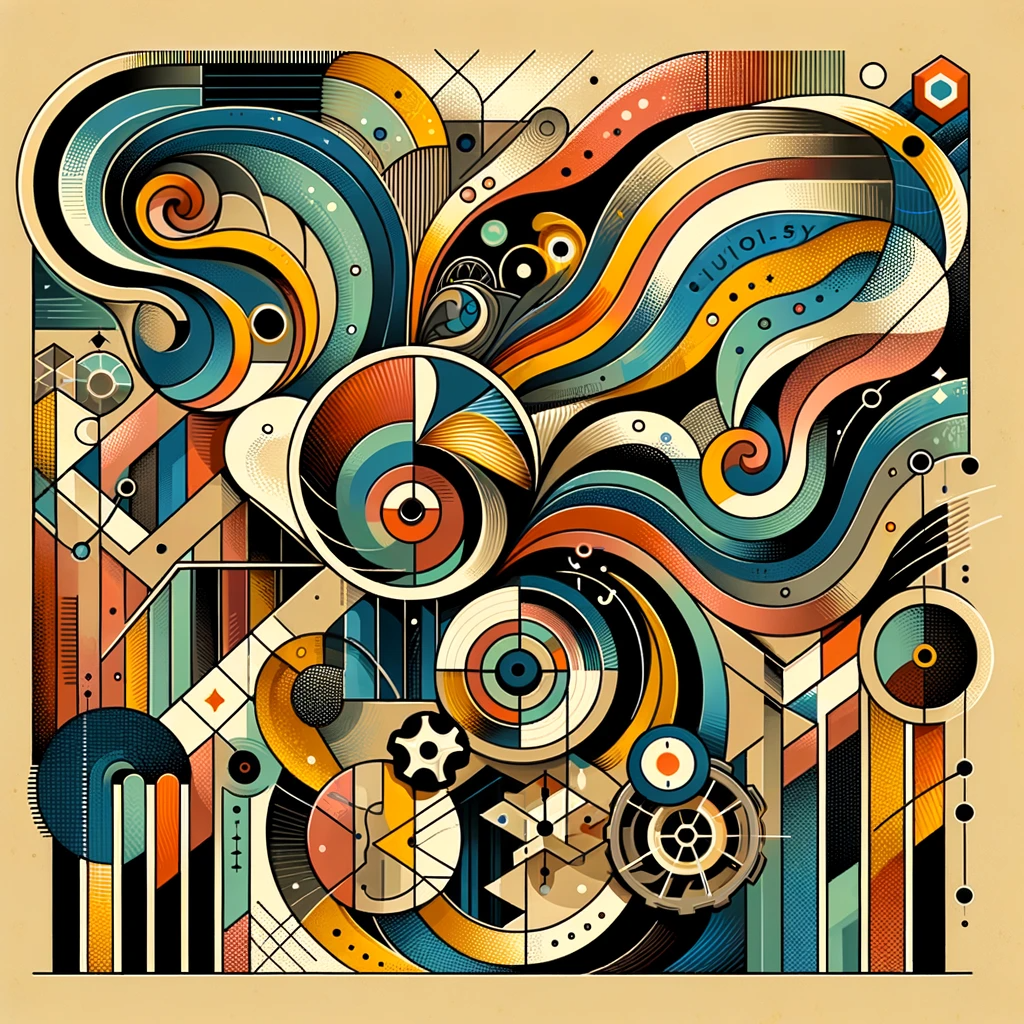This is a complex piece of modern abstract art set against a beige, almost gold background. The artwork features a dynamic interplay of geometric shapes and flowing swirls in a palette of dark blue, white, black, gray, yellow, orange, red, rust, gold, and various greens. At its center, the focal point, about six orbs display intricate swirls of color lines, adding depth and movement. Orthogonal lines and interlocking gears create a deconstructivist, Picasso-like avant-garde feel, with circles and tubes intersecting in various directions, enhancing the overall complexity and depth of this vibrant piece.